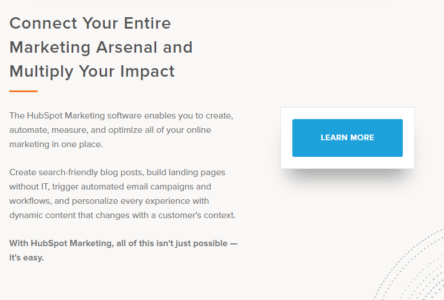The image is a horizontal rectangular graphic that prominently features a message promoting a marketing platform. In the bottom right corner, seven partial arcs made up of small dots create a subtle, eye-catching design element. The main text is set in three boldface lines and reads: "Connect your entire marketing arsenal and multiply your impact." 

Centrally aligned and highlighted by an orange line, the text below elaborates on HubSpot's capabilities, stating: "The HubSpot marketing software enables you to create, automate, measure, and optimize all of your online marketing in one place." 

The following paragraph further details the functionality, explaining how users can "create search-friendly blog posts, build landing pages with IT, trigger automated email campaigns and workflows, and personalize every experience with dynamic content that changes with your customer context."

The next paragraph emphasizes the ease of use: "With Smart Hubs marketing, all of this isn't just possible, it's easy." This line is also set in boldface.

To the right side of the graphic is a white rectangle with a subtle shadow underneath, giving it a three-dimensional appearance. Inside this white rectangle is a blue rectangular button, prominently displaying the call-to-action "LEARN MORE" in bold white capital letters.